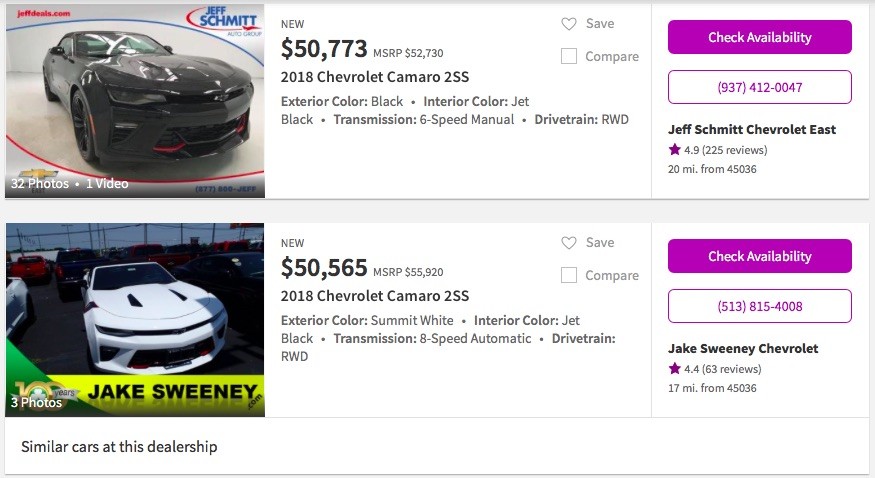### Detailed Caption

The screenshot portrays a segment from a car dealership website, divided into two distinct sections. 

#### First Section:
- **Visual Content**: A front-right side view of a car.
- **Text Information**: 
  - An indicator at the top showcases "32 photos, 1 video".
  - The name "Jeff Schmidt" is prominently displayed.
  - A white banner labeled "New".
  - Pricing details: "New: $50,773" and a manufacturer suggested retail price (MSRP) of "$52,733".
  - Vehicle specifics: "2018 Chevrolet Camaro 2SS".
  - Additional details: Exterior color, interior color, transmission specifications.
  - Options for interaction: "Save", "Compare", "Assist", "Check Availability".
  - Contact information and dealership name: "Jeff Schmidt Chevrolet East".

#### Second Section:
- **Visual Content**: A front view of a white car.
- **Text Information**: 
  - An indicator shows "3 photos".
  - The name "Jake Sweeney" is displayed.
  - Pricing details: "New: $50,565" and an MSRP of "$55,920".
  - Vehicle specifics: "2018 Chevrolet Camaro 2SS".
  - Additional details: Exterior color, interior color, transmission, drivetrain specifications.
  - Options for interaction: "Save", "Compare", "Assist", "Check Availability".
  - Contact information and dealership name: "Jake Sweeney Chevrolet".

Both sections encapsulate detailed vehicle information and provide essential options for potential buyers to interact with the listings or reach out to the respective dealerships.